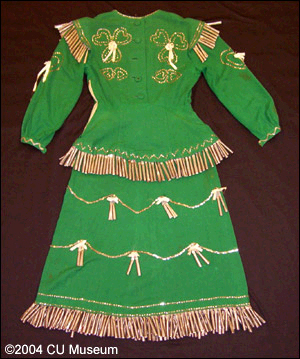The image depicts a low-resolution photograph of a traditional-looking, old-style dress, possibly of Irish origin due to apparent clover motifs. The dress is predominantly green and features intricate embellishments including frilly, gilded fabric or tassels that adorn the shoulders, hips, and bottom edges. The gilded tassels could be made of rope or wood, adding to the dress’s ornate design. Alongside these gilded sections, the dress also has gold embroidery on the chest area, with loops or floral patterns on both the left and right breast, and green buttons fastening the top portion. Further detailing includes ribbon-like designs on the sleeves and front chest section. The dress is laid flat on a black surface, possibly a sheeting or blanket, and the bottom left of the image bears the text "2004 CU Museum," indicating its display location.